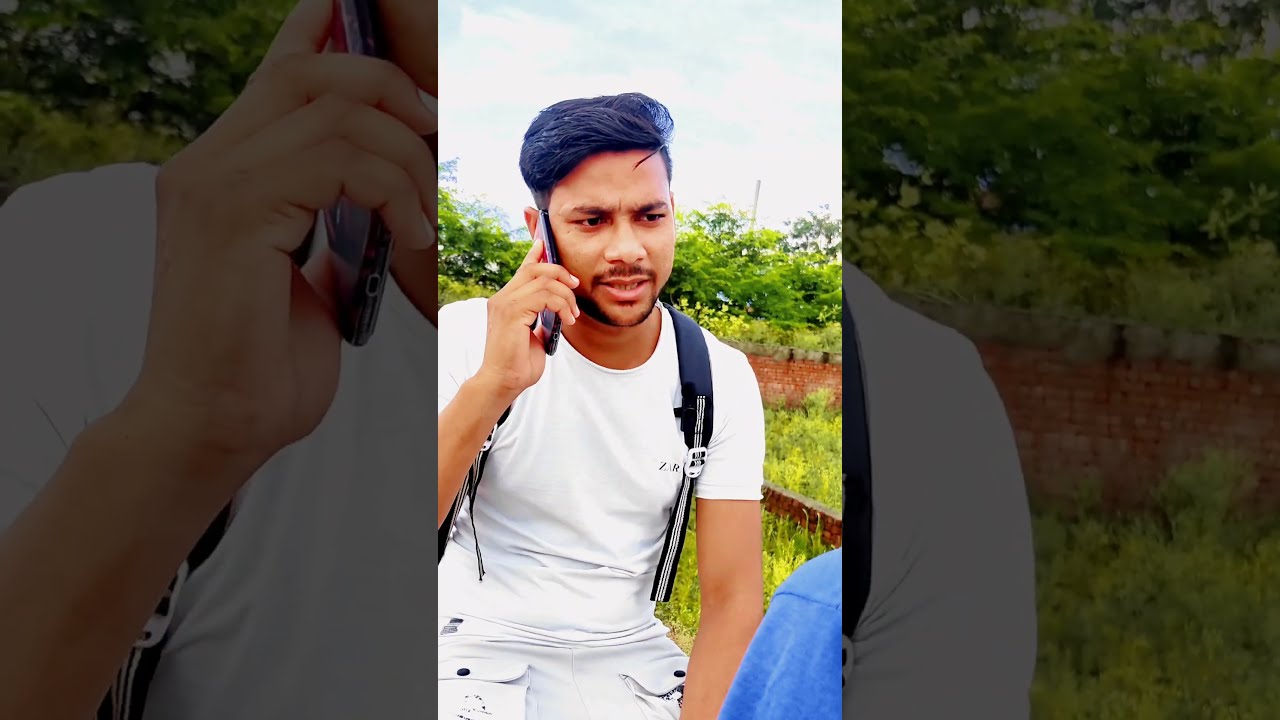In the center of the photo, a man who appears to be of Indian descent is holding a black phone to his right ear while facing slightly towards us. His hair, potentially dyed a purplish color, is styled upwards before curling back in a semi-circle. He has distinct sideburns, a small beard along the jawline, and a mustache framing his mouth, which is slightly open revealing his bottom teeth. He wears a white t-shirt with a logo and off-white cargo pants with large pockets and snaps. A black backpack with padded shoulder straps and black and white tightening pads is slung over his shoulders. His left hand is down, possibly in his pocket or resting by his side. Behind him are green trees and red brick garden beds. The image is presented in a triptych style; the left and right thirds show close-ups of his hand holding the phone and his left shoulder, both with a darker filter, creating a photo-on-photo effect.